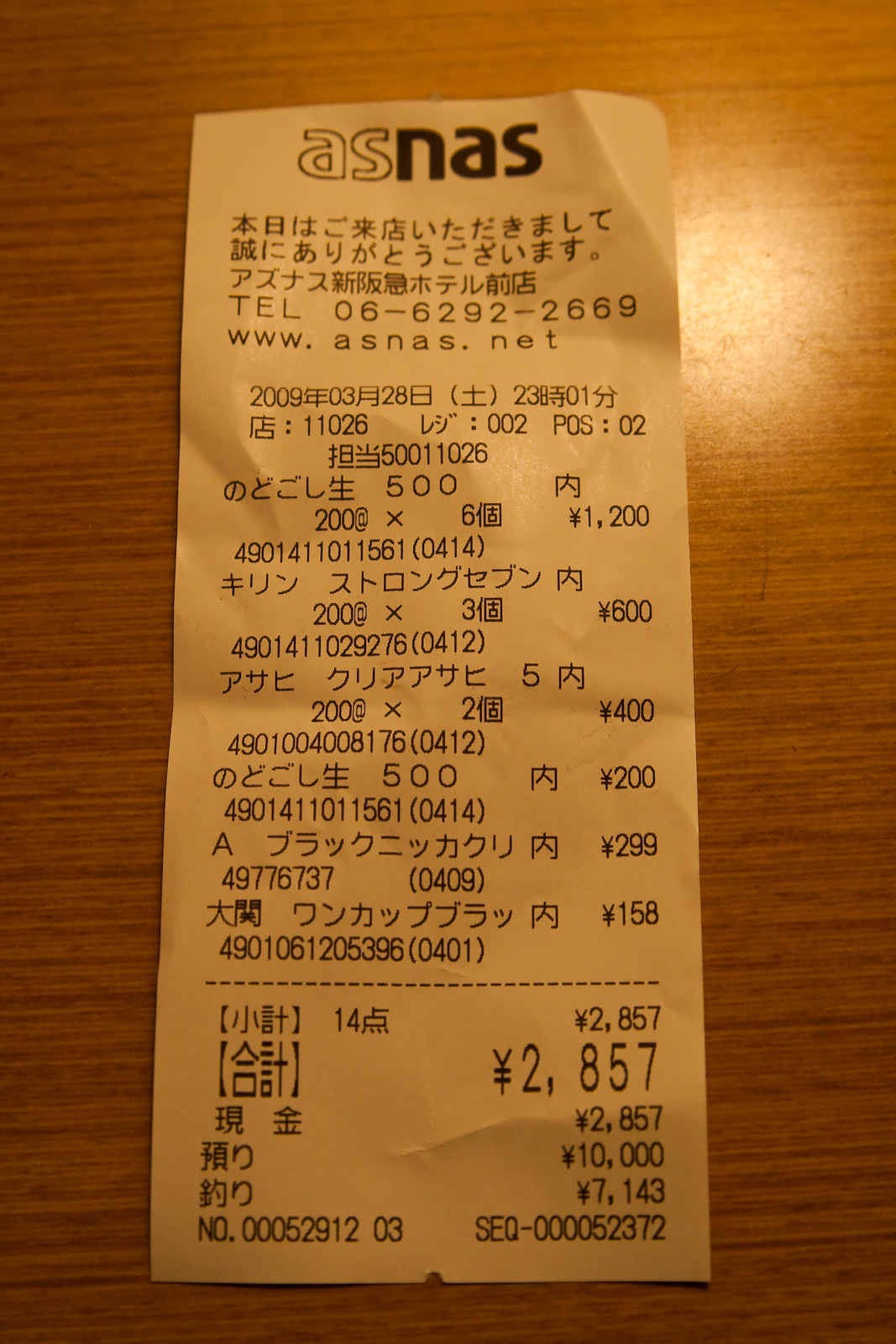A detailed close-up image of a non-American receipt, denominated in Japanese yen, placed on a smooth wooden table. The receipt, issued by ASNAS as indicated at the top, features a white, rectangular format typical of such documents. Below the header with "ASNAS," there is a contact telephone number and a website, www.asnas.net. The receipt is printed primarily in Japanese script, which includes a standard itemized list of purchased goods followed by their corresponding prices: ¥1,200, ¥600, ¥400, ¥200, ¥299, and ¥158, culminating in a subtotal of ¥2,857. Additional items or charges are listed beneath, including amounts of ¥10,000 and ¥7,143, possibly indicating taxes, gratuity, or larger transactions associated with a dining or retail experience. The entirety of the information is presented in a familiar receipt layout, though much of the text remains untranslated. The wood table beneath the receipt is flat and polished, devoid of any noticeable grooves or textures, emphasizing a seamless, single-slab appearance.